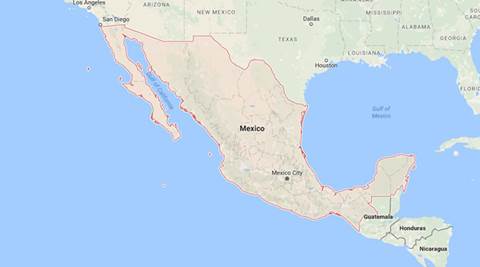This image showcases a detailed map with a focus on Mexico and its surrounding regions, presented in a landscape orientation. The central feature is Mexico, highlighted in a light red color, with clear delineations of its borders. The map designates Mexico's capital, Mexico City, with a small gray dot, and labels the country with "Mexico" in bold black text.

The map extends beyond Mexico to include parts of its neighboring countries. To the south, it displays three Central American countries in standard green map coloring: Guatemala, Honduras, and Nicaragua. To the north, it features the bordering U.S. states. Arizona, prominently labeled, includes the cities of Los Angeles and San Diego. New Mexico lies to the right of Arizona, followed by Texas, which prominently marks Dallas and Houston.

Additionally, the map captures other Southern U.S. states: Louisiana, Alabama, Georgia, Florida, South Carolina, and Mississippi. The oceans flanking Mexico on both the left and right sides are depicted in light blue, providing a stark contrast to the landmasses.